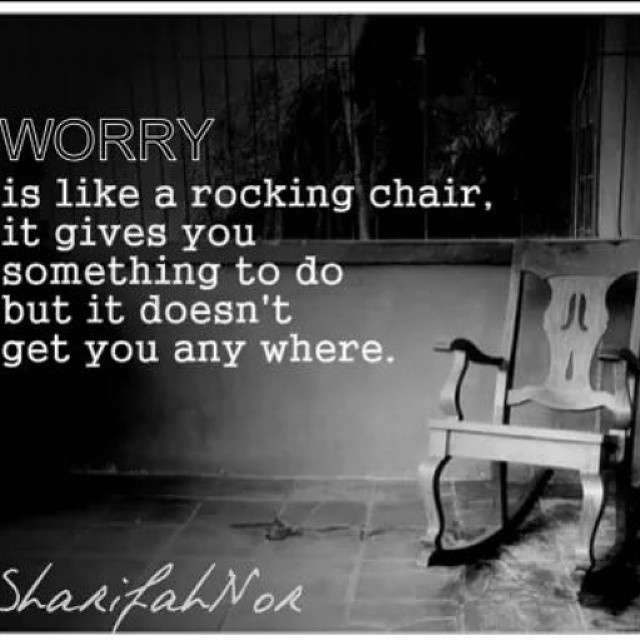The image features a black and white photo of an old, rustic room with rough tile floors, a white-washed wall, and a window framed by bars. In the right-hand corner, there's an empty rocking chair made of wood with a unique back design, adding to the vintage feel of the scene. Superimposed prominently in the image is a quote in large, outlined letters that reads "Worry" followed by the words "is like a rocking chair; it gives you something to do but it doesn't get you anywhere," written in white font. The attribution at the bottom left corner, though slightly hard to read, appears to be a cursive signature, likely "Sharifa Noor."